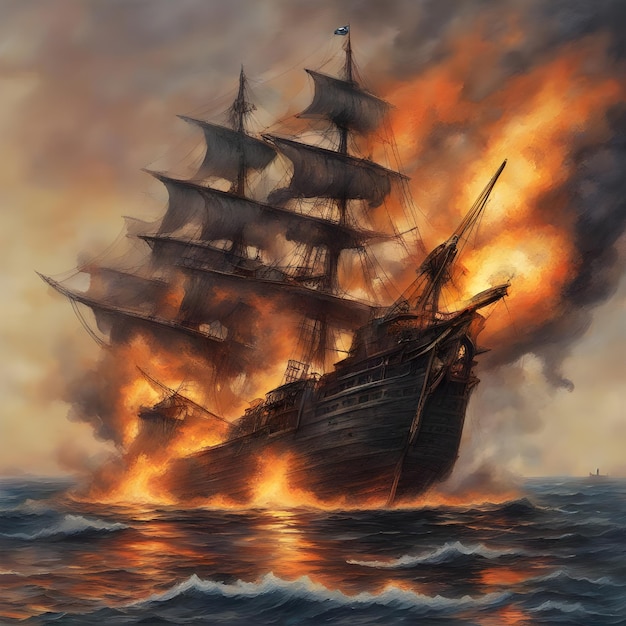This captivating painting depicts an old-fashioned schooner, possibly a pirate ship, engulfed in fierce flames. The vessel, crafted from dark brown wood, features two tall masts adorned with numerous white sails. The inferno is concentrated at the back of the ship, with vivid orange and yellow flames curling up into the dark sky, which transitions to black with hints of tan and brown due to smoke. The ocean below is an almost black blue, with white caps suggesting tumultuous waves reflecting the fire's glare. In the distant right edge of the painting, another vessel is faintly visible. The dramatic scene, marked by swirling dark clouds and smoke in the sky, combines a sense of chaos and beauty, making the painting a striking visual narrative.